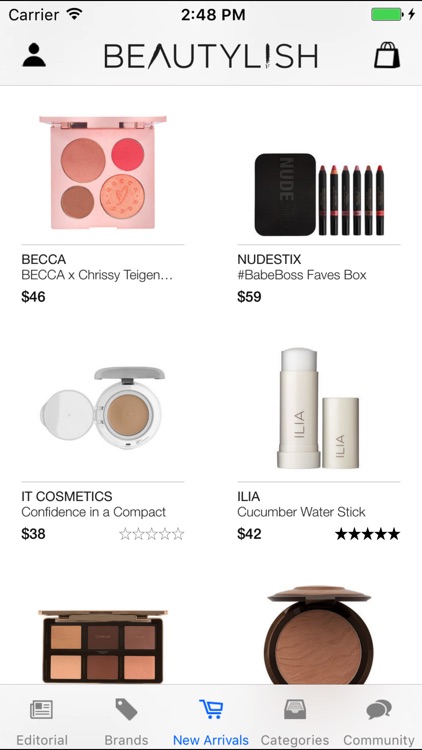In this image, we see a mobile app interface named "Beauty Lash." The app features a stylized logo where the "A" in "Beauty" is depicted as an unfinished triangle, and the "I" in "Lash" is represented by an exclamation point.

At the very top of the screen, on the left, there is a "Carrier" label along with a Wi-Fi icon. The time is displayed prominently in the center as "2:48 PM." On the right, we see a fully charged battery icon.

Directly below this top bar, on the left, there is a profile icon followed by the app name in the center and a shopping bag icon on the right. 

In the main content area, there are six featured makeup products listed: 

1. Becca - $46
2. Nudestix - $59
3. IT Cosmetics - $38
4. ILIA - $42, which has a five-star review
5. & 6. Two unnamed products: one is a palette with six colors on the left, and the other is a single circular color on the right.

At the bottom of the screen, there are five navigational categories from left to right: "Editorial," "Brands," "New Arrivals," "Categories," and "Community." The entire interface, excluding the topmost information bar, has a clean white background.